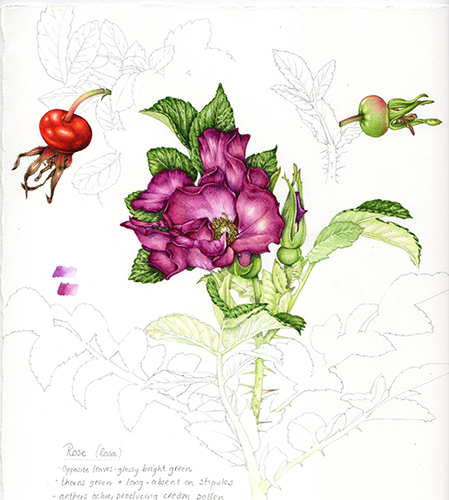This image is a detailed ink drawing and partially colored illustration of a rose. Central to the artwork is a rose in full bloom, with petals in shades of purple and pink. Surrounding the bloom are vibrantly green leaves and a stem, partially filled in with color. The rest of the rose's structure, including additional stems and leaves, mostly remains as delicate black ink outlines awaiting color.

Alongside the main rose, there are other elements incorporated into the drawing. On the left side, there is a red radish-like object, perhaps representing a flower or seed. On the right, a similar element is depicted in green. At the upper portion of the image, above the rose, outlines of leaves and potential flower buds or fruits, resembling small tomatoes or berries, are drawn but not filled in.

The lower part of the image contains some textual annotations in light gray script, challenging to decipher. The visible text includes the words "rose" and "Rosa," along with fragments of further descriptions, such as "bright green," "thorns green," and references to various plant parts like "staples" and "pollen," suggesting detailed botanical notes.

Overall, the artwork merges the precision of vintage botanical illustration with a work-in-progress aesthetic, showcasing the blend of completed color sections and intricate line work awaiting final touches.